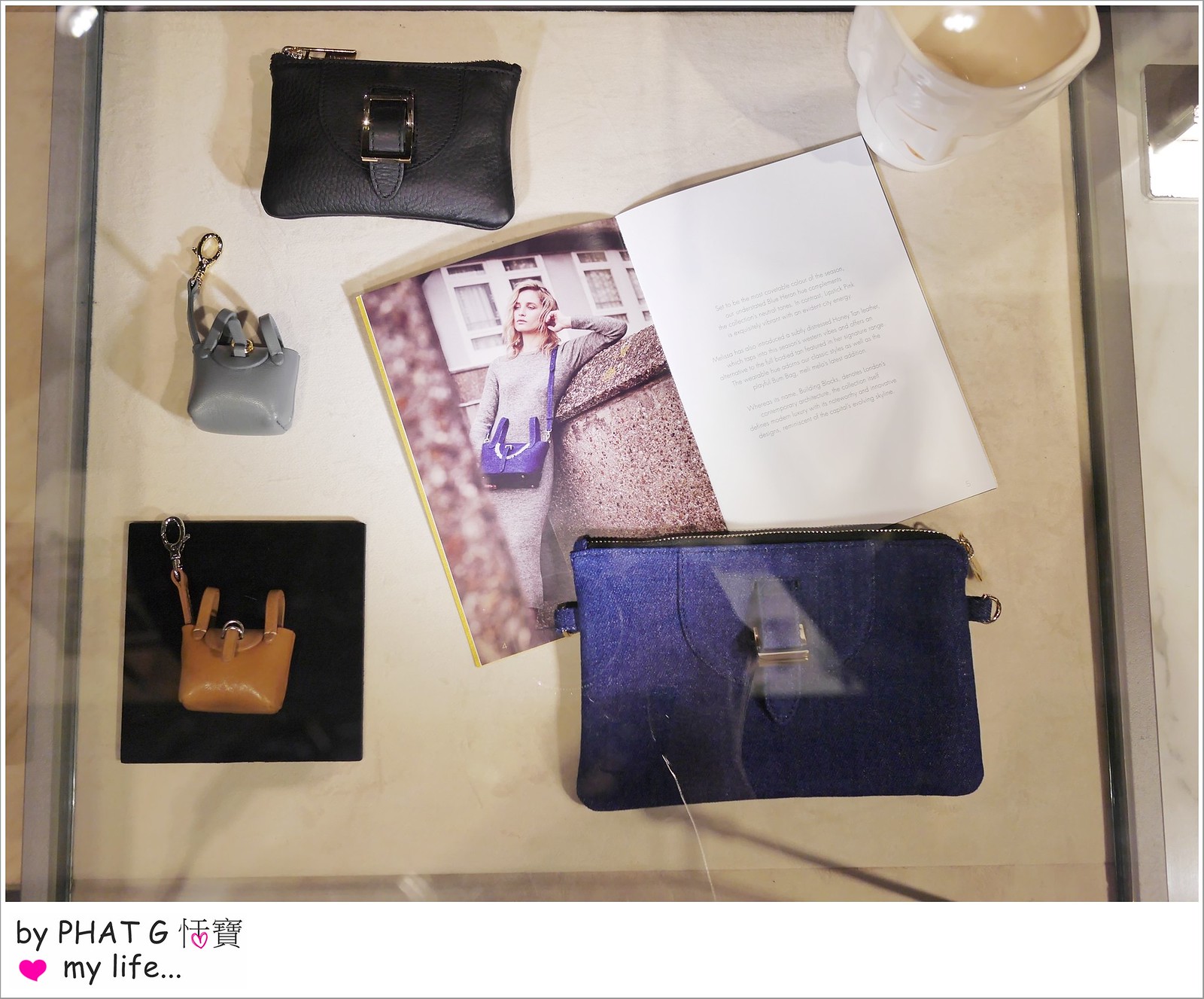The photograph captures a top-down view of a meticulously arranged display on a light tan table, resembling a personal showcase. At the top left corner sits a small black leather change purse with a buckle. To its right is a tiny gray coin purse with a clasp, and beneath it, a similar beige coin purse situated on a square black fabric. Both small purses have keychain clips. The top right corner features an off-white ceramic cup with the semblance of a face etched into it. Centrally positioned in the layout is an open magazine. The right page of the magazine contains text, while the left page displays a photograph of a blonde-haired woman in a long, gray, long-sleeve dress, posed elegantly against a wall with her elbow resting on it and her hand touching her face. She wears a blue or purple purse draped over her left shoulder, resting in front of her body. In the foreground, partially covering the magazine, lies a larger blue clutch bag without straps. At the bottom left of the image, near the model's page, text reads "By Phat G," accompanied by a pink heart and the words "My Life" alongside some Asian symbols, hinting at a social media post context. The arrangement is thoughtfully designed, creating an aesthetic and personal display reminiscent of cherished items exhibited under glass.